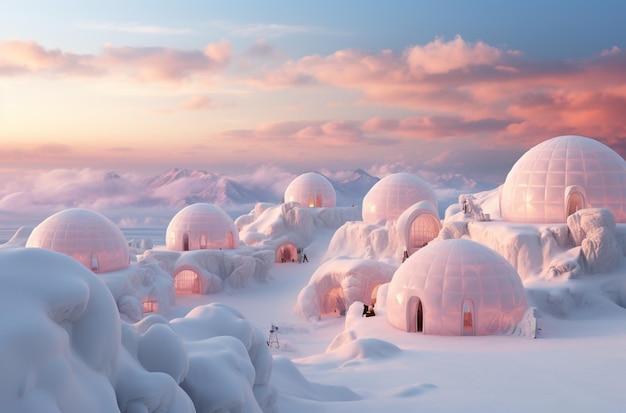The image is a computer-generated graphic depicting a serene Arctic landscape populated by a small community of igloos. Each igloo, pearl white with a subtle pinkish hue at its base, rests atop individual ice-covered rocks, presenting a scene reminiscent of a neighborhood. The igloos are meticulously crafted, resembling small homes with visible lighting details on their sides. In the distance, imposing snow-covered mountains frame the scenery, their peaks veiled by light clouds tinged with a delicate pink shade. A few tiny figures can be seen outside the igloos, emphasizing the scale against the expansive backdrop. The sky above is a soft gradient, transitioning from blue to hints of a setting sun's glow, adding to the tranquil and picturesque ambiance of this Arctic community.